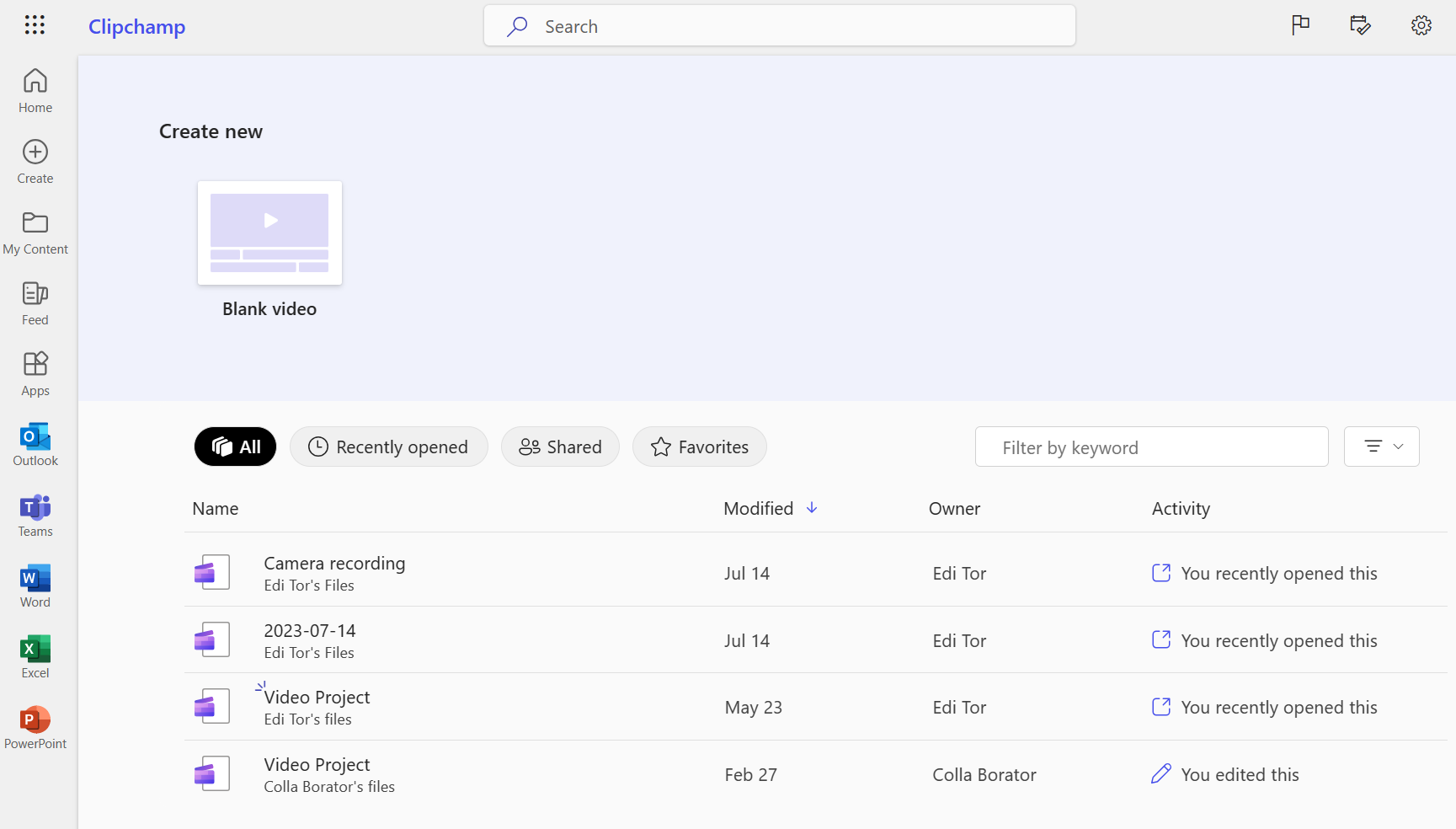The image features a user interface of a digital application, presumably a video editing platform, with a prominent gray rectangular menu on the left side. At the top left corner of the interface, the word "Clipchamp" is clearly displayed. Below this, a vertical column of eight icons is presented, with the first five icons in black representing "Home," "Create," "My Content," "Feed," and "Apps." The subsequent three icons are in blue, labeled "Outback," "Teams," and "Word," followed by a green icon labeled "Excel," and a red icon labeled "PowerPoint."

Beneath the "Clipchamp" label, there is a lighter gray rectangle containing the black text, "Create new." Adjacent to this is a small white rectangle with a gray interior and a smaller rectangle inside, resembling a little brick wall. At the bottom of this darker gray section, there is text reading "Blank Video," suggesting an option to start a new blank video project.

Further down, user options are presented in button form, starting with a black button labeled "All" followed by gray buttons labeled "Recently Opened," "Shared," "Favorites," and "Filter by Keyword."

To the right, four vertical columns organize the content. The first column, titled "Camera Recording," lists video projects dated "2003 7-14." The second column, labeled "Modified," presents various modification dates: "July 14th," "May 23rd," and "February 27th." The third column, titled "Owner," indicates the project owners as "EDITOR" for the first three entries and "COLLABORATOR" for the last entry. The fourth column, titled "Activity," notes actions with entries reading, "You opened this," "You recently opened this," and "You edited this."

Overall, the detailed layout and organization of this interface provide a streamlined way to navigate various content management features.